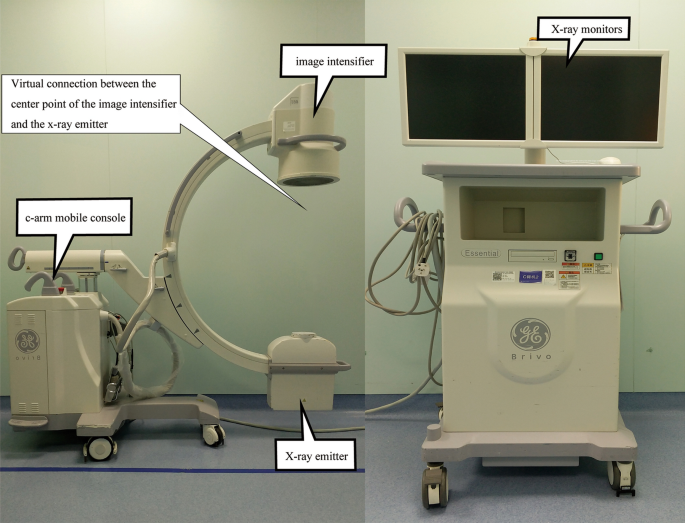The image depicts two side-by-side pictures of a portable x-ray machine, featuring detailed part labels. The left image provides a side view of the GE-manufactured mobile x-ray unit. It shows a C-arm apparatus with an image intensifier at the top and an x-ray emitter at the bottom, both mounted on vertically stacked arms. The label indicates a "virtual connection between the center point of the image intensifier and the x-ray emitter." The C-arm rotates to enable taking x-rays from various angles while the patient stands between the intensifier and emitter. Adjacent to this setup is the mobile console, consisting of two x-ray monitors mounted on a stand, which can be positioned separately for ease of use. The equipment is cream-colored and includes the brand name "Brivo." The right image portrays a disconnected mobile console with two x-ray monitors labeled "x-ray monitors," emphasizing the portability and adaptability of the system for hospital use. The entire assembly, equipped with wheels and labeled components, facilitates efficient patient testing and diagnostic imaging.